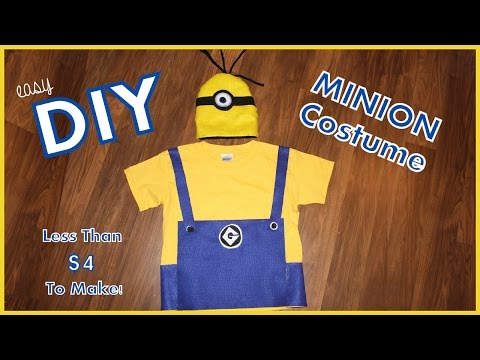This image displays a detailed DIY minion costume layout. The background is a wooden surface bordered by yellow on the sides and black on the top and bottom. In the center, there is a laid-out costume consisting of a yellow shirt and blue suspenders. The shirt features the iconic 'G' logo from the Minions franchise. Accompanying the shirt is a yellow beanie with a single black eyeball detailed in the middle, surrounded by black bands extending to the sides. The text "Easy DIY Minion Costume" is prominently displayed with "Easy" in cursive and "DIY" in white letters on a blue background. "Minion Costume" is written in blue text with a white border. Additionally, the bottom left corner of the image reads "Less than $4 to make", indicating the low cost of the project. The layout highlights an accessible, cost-effective guide for creating a fun minion costume.